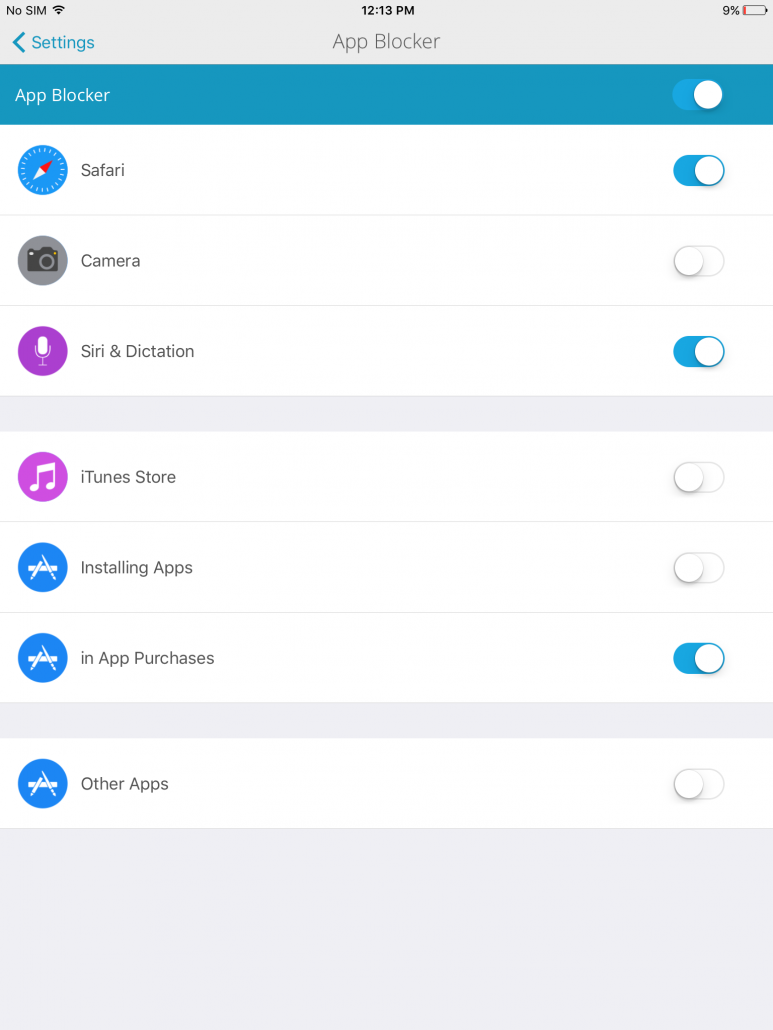Here's a detailed and cleaned-up caption for the image:

"The screenshot displays the settings page of a mobile device at 12:23 PM, indicated by the status bar at the top which also shows 'No SIM' and a critically low battery at 9%, marked by a red icon. Below the status bar, the settings page title is prominently displayed. Directly underneath, the 'App Blocker' is listed with a blue toggle indicating it is enabled. Next, 'Safari' also has its toggle switched on. 'Camera' follows, with its toggle turned off. 'Siri and Dictation' is enabled, while the 'iTunes Store' and 'Google Apps' are both disabled. Lastly, 'In-App Purchase' is toggled on, and 'Other Apps' remains off."